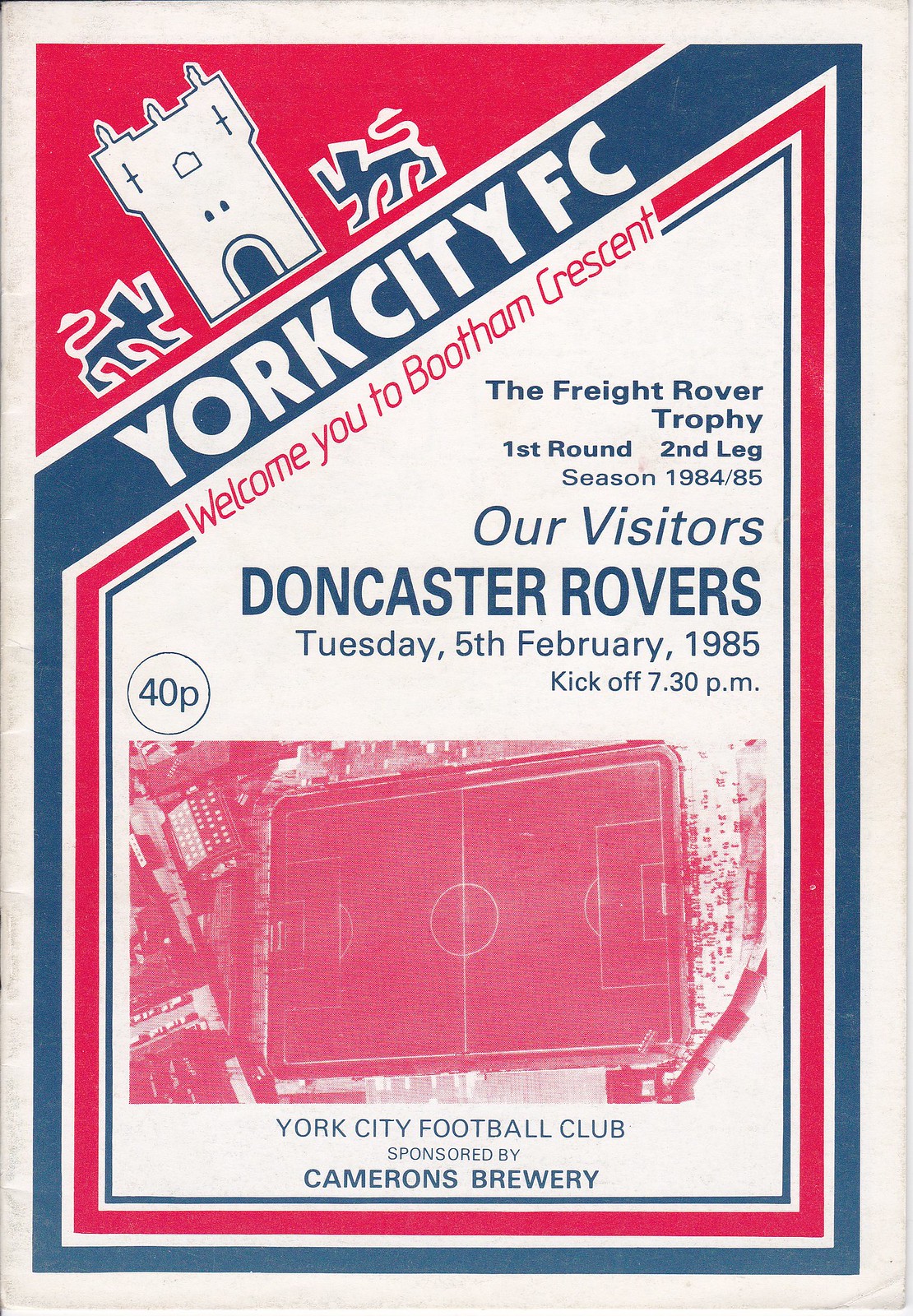This is a detailed picture of a soccer match program or flyer from York City FC. The background is predominantly white with distinct red, blue, and white borders framing the content. At the top left corner, there is a triangular depiction of a white castle with a blue arched door, flanked by blue lions, symbolizing something significant about the town. Below this, in large, bold white letters on a blue background, it says "York City FC." In a slanted red print, it reads, “Welcome to Bootham Crescent,” presumably the name of the stadium. Following that, in blue print on a white background, it mentions “The Freight Rover Trophy, first round, second leg, season 1984-85.”

Further down, the text continues to highlight event details: “Our visitors: Doncaster Rovers, Tuesday, 5th of February, 1985, kickoff 7:30 p.m.” Additionally, to the left, there’s a circular emblem stating “40p,” indicating the price. Below this, an aerial depiction of a soccer pitch in red is displayed, appearing as if taken from above. The bottom text reads “York City Football Club, sponsored by Cameron's Brewery.” The overall design is vibrant with a combination of blue, red, and white elements, contributing to its visual appeal and clarity.